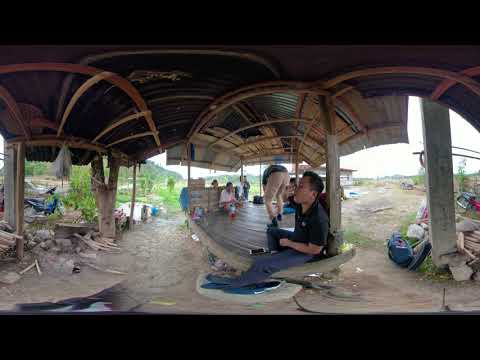The image depicts a group of men working in a partially constructed building, possibly installing flooring. The location appears to be an impoverished area with a cluttered and disorganized environment. The building itself is unfinished, lacking walls but featuring a dark brown roof supported by gray concrete columns and wooden rafters. The men, one in a white shirt and blue jeans, another in tan pants and a dark shirt, and a third in a black shirt and blue jeans, are engaged in tasks such as bending over to install soft brown plank flooring and hammering it into place.

The background shows a scenic landscape with light tan sandy roads, patches of green grass, and sloping hills that form a distant mountain range. Trees and grass provide a lush contrast to the otherwise brown and dirt-filled ground. A blue vehicle is visible on the left side of the image. The overall atmosphere suggests a setting in an Asian country, marked by its bamboo-like ceiling structure and the presence of an Asian man who is resting and possibly eating amidst the clutter. The sky is overcast, lending a muted, white hue to the backdrop.